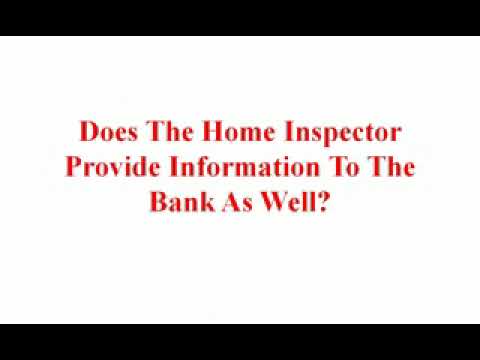This image features a question displayed prominently against a plain white background, bordered by solid black horizontal bars at the top and bottom. The centered text, written in bold and dark red Times New Roman font, spans three lines and reads, "Does the home inspector provide information to the bank as well?" The image appears to be a low-resolution slide from a presentation, possibly related to home inspections, with noticeable digital compression artifacts affecting the clarity of the text.